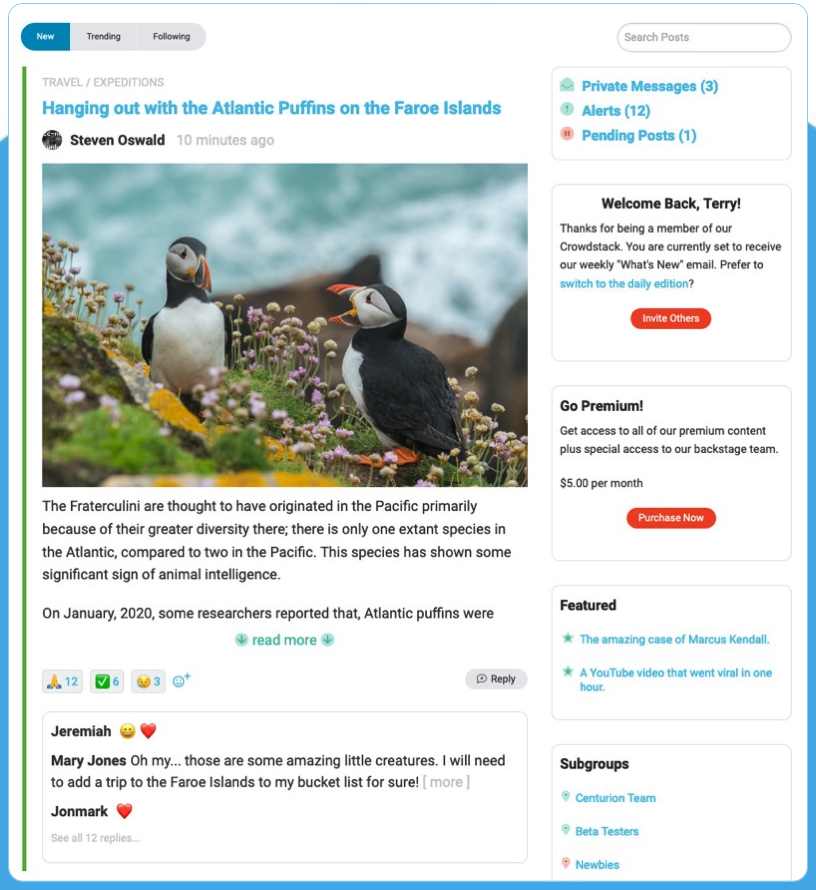**Title: Exploring the Faroe Islands with Atlantic Puffins**

**Detailed Image Description:**

**Format:** Vertical rectangular image.

**Border:** The image features a light turquoise border across the top horizontally, which slightly extends down the right and left sides. This border transitions into a thick, bolded line which continues three-quarters of the way down the left side, across the bottom, and then three-quarters of the way up from the bottom on the right side.

**Header:** At the very top, there is an oval horizontal section divided into three parts. The left part says "NEW" in a white font on a turquoise background. The middle and right parts say "TRENDING" and "FOLLOWING" respectively, both with a gray background and black fonts.

**Subheader:** Below the oval section, in a light gray font and all capitalized, it says "TRAVEL / EXPEDITIONS." Underneath this, in bold turquoise font, it reads: "Hanging out with the Atlantic puffins on the Faroe Islands."

**Author and Timestamp:** Further down, it mentions "Stephen Oswald" in black text, followed by "10 minutes ago" in gray text.

**Main Image:** A horizontal rectangular image showing two Atlantic puffins facing each other. One puffin is positioned in the lower right corner looking toward the upper left, while the other faces down towards the lower right. Both birds have black backs and heads, white stomachs, and yellow-orange beaks. They are amidst green grass and small purple flowers.

**Article Excerpt:** Below the image, black text reads: "The Fraterculini are thought to have originated in the Pacific primarily because of their greater diversity there. There is only one extant species in the Atlantic compared to two in the Pacific. The species has shown some significant signs of animal intelligence. On January 2020, some researchers reported that Atlantic puffins were..." The excerpt ends with a "READ MORE" link in green text accompanied by a down arrow.

**Comment Section:** At the bottom of the page, a user named "Jeremiah" (in bold with a smiley face and heart) comments: "Oh my, those are some amazing little creatures. I will need to add a trip to the Faroe Islands on my bucket list for sure." Another user, "Mary Jones" in bold text, shares similar sentiments. "John Mark" also comments with a red heart emoji.

**Sidebar Information:**

- **Top Left Corner:** In turquoise text, it reads: "Private messages 3, Alerts 12, Pending posts 1."
- **Welcome Message:** "Welcome back Terry" in black bolded font, with a smaller, non-bolded font reading: "Thanks for being a member of our Crowd Stack. You are currently set to receive our weekly What's New email. Prefer to" in turquoise text, followed by "switch to the daily edition."
- **Premium Content Box:** Next, a black bolded font reads: "GO PREMIUM," with smaller text underneath: "Get access to all of our premium content plus special access to our backstage team for $5 a month." This is followed by a red heart and a reddish-orange horizontal area with white lettering that reads: "Purchase now."
- **Featured and Subgroups:** Below this, there are two more sections. The first, titled "Featured," includes "The amazing case of Marcus Kendall and a YouTube video that went viral in one hour" in turquoise text. The second, titled "Subgroups," lists "Centurion team, Beta testers, and Newbies" in turquoise.

**Vertical Line:** Along the thick vertical line on the left edge, there's also a green vertical line starting slightly lower than the top edge and almost reaching the bottom, but not quite touching.